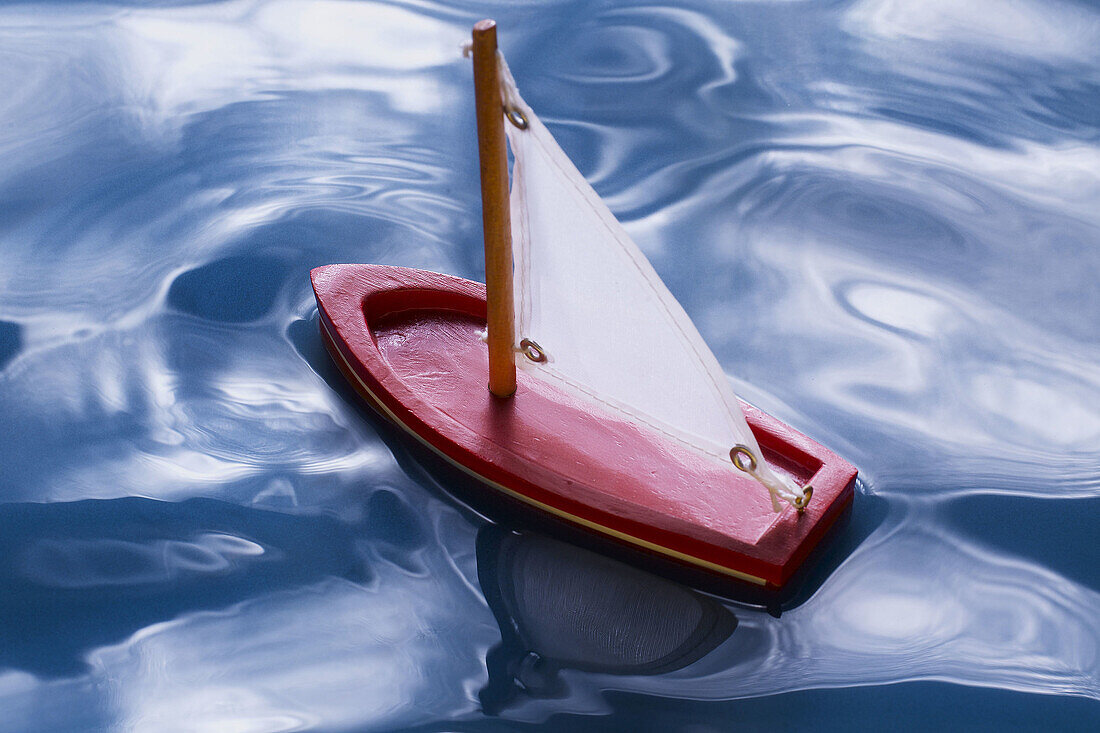This image features a detailed, hand-carved wooden toy sailboat, painted vividly in red with a distinct yellow stripe along its outer edge, floating on rippling blue water. The boat itself is small, resembling a canoe with a flat back and an indented top, suggesting a space where one might imagine placing a tiny figure. At its center, a light brown wooden mast rises, supporting a triangular white sail made of fabric. The sail is fastened to the mast and the boat with strings running through gold-colored grommets at each corner, creating the impression of a functional sail fluttering in a gentle breeze. The water, though featuring pronounced ripples and light reflections, remains ambiguous—its striking clarity and detail make it unclear whether the image is a photograph, a painting, or a piece of digital art. The scene captures a serene and timeless image of the miniature vessel poised in its watery setting.